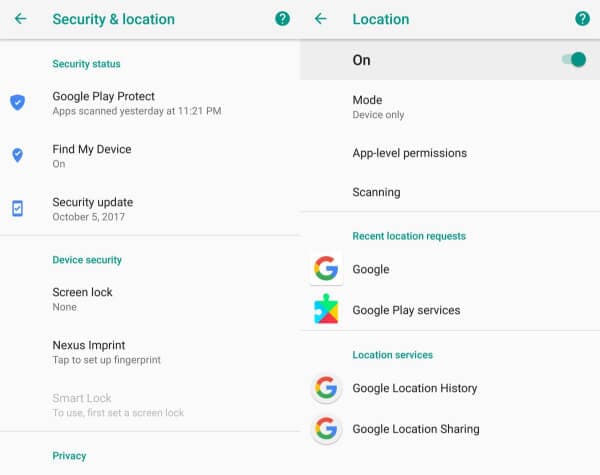The image comprises two side-by-side screenshots depicting settings on a mobile device. 

**Left Screenshot:**

- **Header**: The top header contains green text reading "Security & location" alongside a green back arrow to the left. The background in this section is light grey with an underline separating the header from the rest of the content.
  
- **Sections and Items**:
  - **Security Status**: This section starts with smaller green text that reads "Security status" and features three items beneath:
    - Google Play Protect
    - Find My Device
    - Security Update
  - **Device Security**: Below the above-mentioned items, a new section titled "Device Security" in green text includes:
    - Screen lock: None
    - Nexus Imprint
    - Smart Lock
  - **Privacy**: At the bottom of the left screenshot is another section titled "Privacy".

**Right Screenshot:**

- **Header**: The top header showcases the word "Location."
  
- **Sections and Items**:
  - **Toggle Button**: Directly below the header is the word "On," accompanied by a green toggle button indicating that location services are enabled.
  - **Additional Options**: The screenshot mentions further options: Mode, Level, Permissions, and Scanning.
  - **Recent Location Requests**: This section lists the most recent location requests made by apps on the device.
  - **Location Services**: The final section in the right screenshot is titled "Location Services."

The background of both screenshots prominently features a light grey color scheme, consistent with standard settings interfaces.